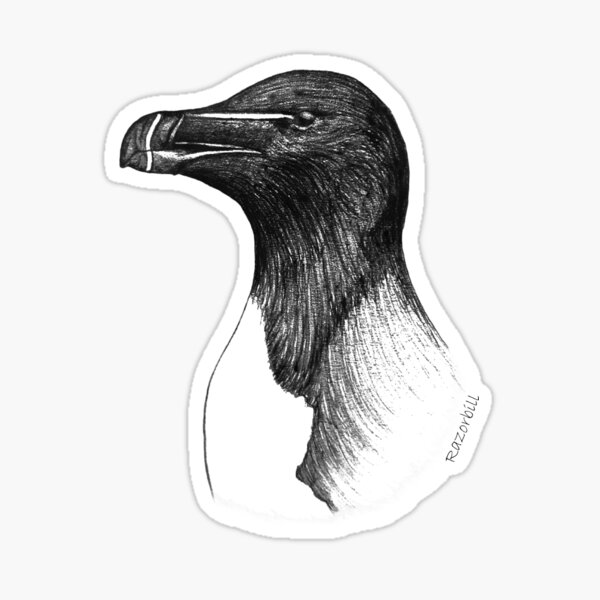The image features a detailed cardboard cutout of a bird's head set against an off-white or cream-colored background. The bird appears to be a black-and-white sketch with intricate details. Surrounding the sketch, a white border creates the appearance of a cutout, enhanced by a subtle shadow on the background for a three-dimensional effect. Notably, the cutout is perforated, adding an interesting tactile element.

The bird, identified as a Razorbill, has a striking black head contrasted by a lighter, more sparsely shaded neck, indicating a different feather coloration. Its distinctive beak is rounded at the top and tapers to a point, adorned with white lines on the lower beak and an additional white line extending from its dark eye to the top beak, crossing the nose area. The bird's eye is noticeably dark, adding depth to the sketch. At the bottom right corner of the cutout, the name "Razorbill" is printed in black letters, providing a clear identification for the viewer.